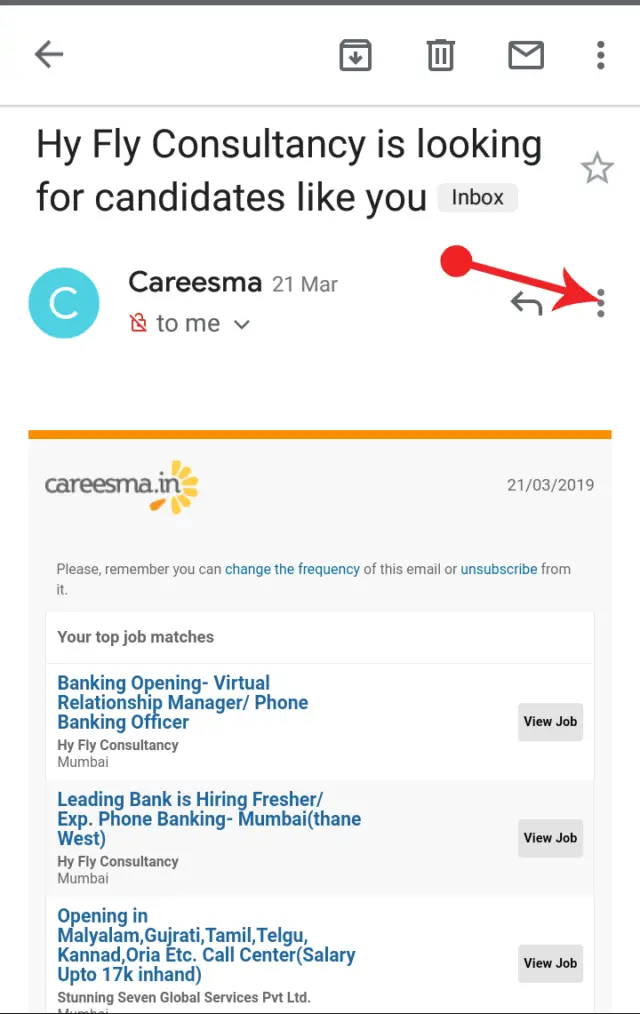**Screenshot Description: Hi Fly Consultancy Job Email**

The screenshot displays a notification email from Hi Fly Consultancy, a recruitment agency. The top section features typical email navigation elements: a back arrow, a download button, a trash can, an envelope, and a triple-dot vertical menu. The sender information includes a "Hi Fly Consultancy" label (spelled "Hi Fly" where "Hi" is stylized as "H-Y") and the tagline "Hi Fly consultancy is looking for candidates like you." Adjacent to this, the term "inbox" is displayed with a star icon to its right.

Centered below, a light blue circle with a "C" inside it identifies the email as originating from "charisma," spelled "C-A-R-E-S-M-A," dated 21st January. The email is addressed "to me." Additional navigation includes a return arrow and another vertical three-dot menu positioned to the right.

A prominent visual feature is a large red arrow, aimed at the central dot of the vertical menu, starting with a sizable red circle base and flaring at the tip. The rationale for this emphasis is unclear.

Below this, a gold line demarcates the section where "charisma.in" is written with a semi-circle of flower petal-like designs. The email displays the date as 21/03/2019.

The body of the email mentions the ability to change email frequency or unsubscribe. The primary focus highlights top job matches including:
1. **Banking Opening** for a Virtual Relationship Manager and a Phone Banking Officer.
2. A listing titled "Lead Banking is Hiring" seeking Phone Banking Officers in Mumbai, Thane West, applicable to both freshers and those with experience.
3. Job postings in multiple languages (Malayalam, Gujarati, Tamil, Telugu, Kannada, Oriya, etc.) for call center positions offering salaries up to ₹17,000.

Buttons for "View Job" are placed on the right side of these listings. The bottom part of the email contains a thin black bar indicating additional content is available upon scrolling.